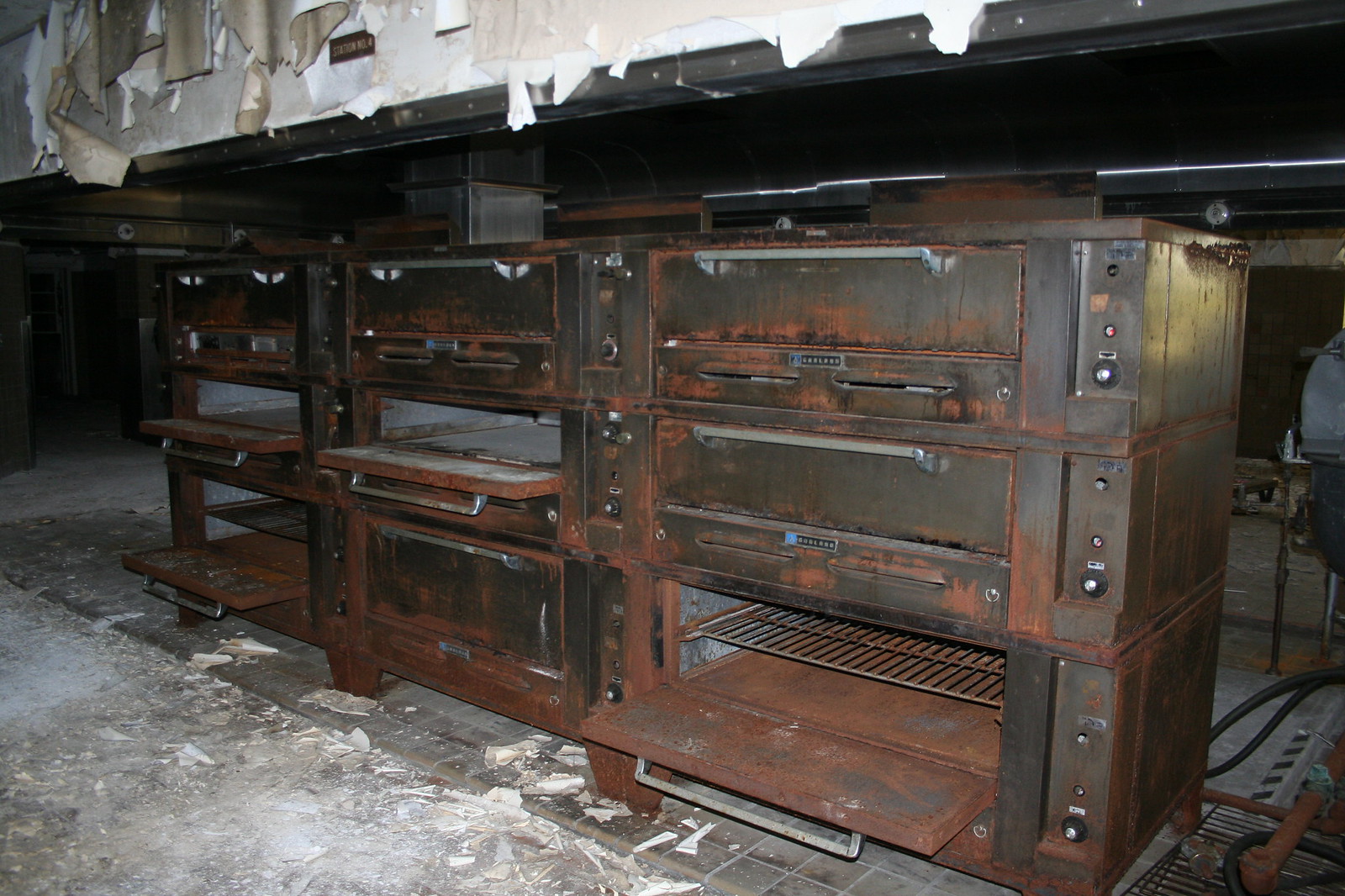This image captures the interior of what appears to be an abandoned and possibly fire-damaged industrial kitchen. Dominating the scene are three stacks of large, rusted professional ovens, arranged three high and three wide. The ovens are heavily corroded, with some doors hanging ajar, allowing a glimpse inside at the rusted racks. The control panels are situated on the right side of each oven, also encrusted with rust. Above the ovens, the walls are clad in peeling wallpaper over crumbling sheet rock, adding to the derelict atmosphere. The floor is a dirty gray, strewn with debris including white plaster and cement chunks. The ceiling is partially exposed, revealing I-beams and ventilation shafts, indicating significant structural decay. A rack and some hoses connected to a tank are visible behind the ovens, further emphasizing the disuse and dilapidation of the space. This scene suggests a long history of abandonment, with no clear indication if it was formerly a restaurant or an industrial food preparation area.